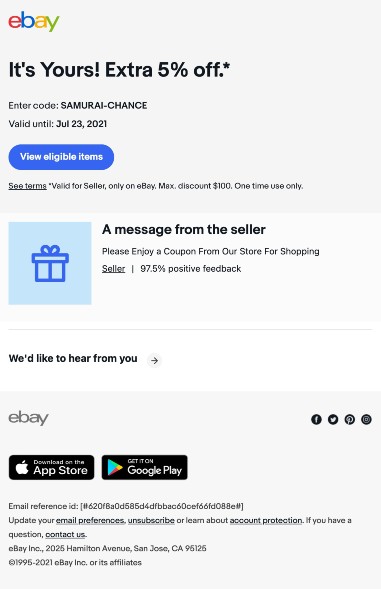The image displays a screenshot of the eBay mobile app. At the top of the page is the iconic eBay logo comprised of a red "e", blue "B", orange "a", and green "y". Just below the logo is a prominent message in black font on a white background, which reads: "It's yours, extra 5% off. Enter code SAMURAICHANCE, valid until July 23, 2021." Following this is a blue button labeled "View eligible items." The terms and conditions state, "See terms valid for seller only on eBay, max discount $100, one time use only."

Further down, the screen displays a message from the seller that invites the user to "please enjoy a coupon from our store for shopping." Accompanying this message is the seller's feedback rating of 97.5% positive. Below this section, there is a button labeled "We would like to hear from you."

Towards the bottom of the screen, on a light gray background, the eBay logo is shown again, followed by two action buttons: one for "Download on the Apple App Store" and another for "Get it on Google Play." The overall orientation and layout of the interface suggest it belongs to a mobile application, likely viewed on a smartphone screen.